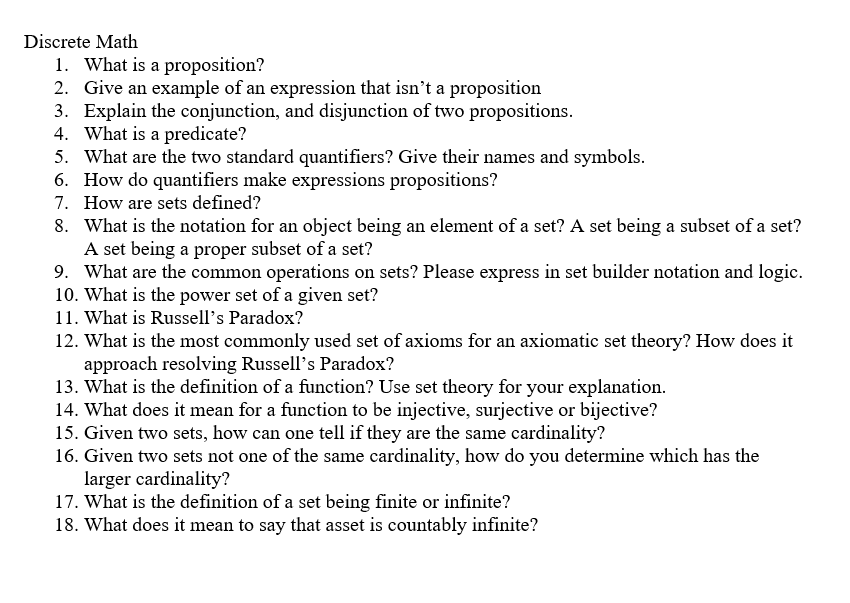The image features a white background filled with numbered sentences concerning discrete mathematics. At the top, the header reads "Discrete Mathematics." The enumerated list runs from 1 to 18 and includes the following:

1. What is a proposition?
2. Give an example of an expression that isn't a proposition.
3. Explain the conjunction and disjunction of two propositions.
4. What is a predicate?
5. What are the two standard quantifiers? Give their names and symbols.
6. How do quantifiers make expressions of propositions?
7. How are sets defined?
8. What is the notation for an object being an element of a set, a set being a subset of another set, and a set being a proper subset of another set?
9. What are the common operations on sets? Please explain in set builder notation and logic.
10. What is the power set of worth?
11. What is the power set of a given set?
12. What is Russell's Paradox?
13. Define what it means for a set to be finite or infinite.
14. Explain what it means for a set to be countably infinite.

The content focuses on fundamental concepts and questions in discrete mathematics, detailing logical and set theoretical notions.